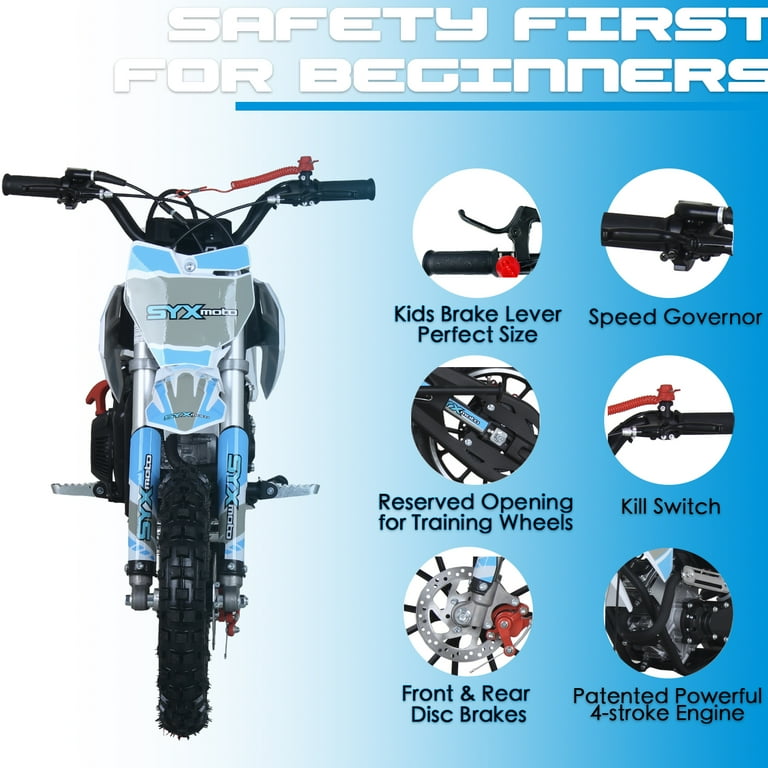The image is a square-shaped advertisement for a children's dirt bike set against a background that transitions from blue on the right to white on the left. On the left side of the image, the dirt bike is positioned head-on, showcasing its features. It boasts black handlebars and prominently displays the brand name "SYX Moto" on a front shield, which is adorned with graphic designs in silvery gray and blue. The bike's nubby front tire is complemented by light blue and silver front forks, also marked with the company's name.

Across the top of the image, large white letters spell out "Safety First for Beginners". Below this title, six close-up detail photos are enclosed in white circles, distributed in two rows. The top row includes:
1. **Kid's Brake Lever - Perfect Size**: Demonstrating the brake lever optimized for children.
2. **Speed Governor**: Showcasing a feature that controls the bike's speed.

The second row features:
3. **Reserved Opening for Training Wheels**: Indicating the bike's capability to accommodate training wheels.
4. **Kill Switch**: Highlighting a red kill switch for safety, previously mistaken for a throttle.

The final row presents:
5. **Front and Rear Disc Brakes**: Featuring images of the bike's perforated metal disc brakes and their corresponding clamps.

On the right side of the image, text highlights a "Patented Powerful Four-Stroke Engine", accompanied by a photograph of the black engine.

Overall, this detailed and visually engaging advertisement emphasizes both the safety features and the advanced components of the SYX Moto dirt bike, making it an appealing choice for young beginners.